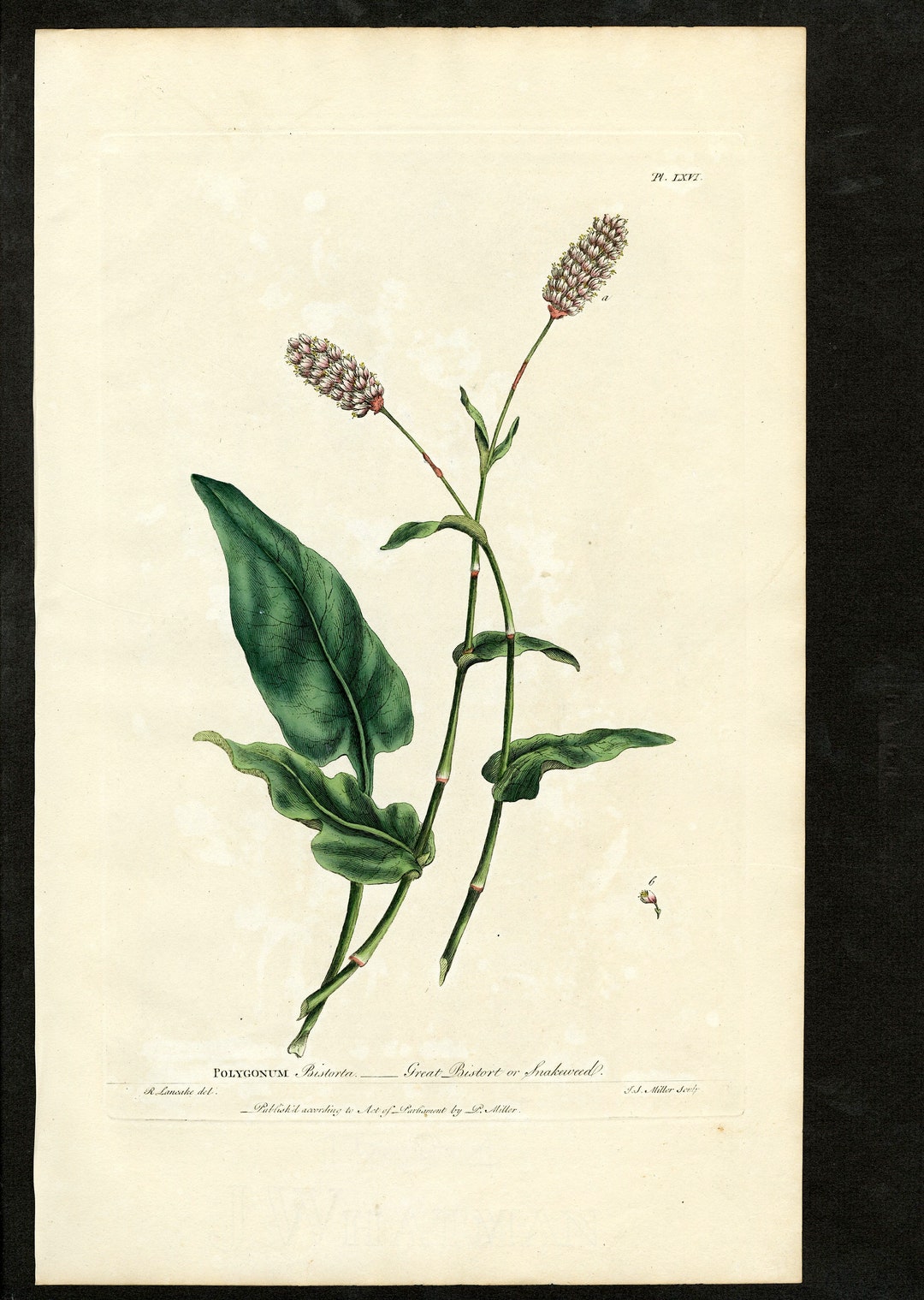This detailed vintage botany illustration features an off-white background with three prominent green plant stalks. Rendered in watercolor, the intricate details highlight the botany study's age and artistic craftsmanship. Each of the three stalks is characterized by a semi-thick, light green stem and large, wavy, dark green leaves. Notably, the central stem is adorned with blooming flowers that are cone-shaped, predominantly purple with white accents, and have pink bases. The first stem displays a significant leaf jutting out to the left, while the following two stems have multiple leaves that droop downward. At the bottom of the illustration, partially faded but discernible, is the name "Polygonum bistorta," commonly known as grape bistort or shakeweed, along with a fancier font indicating "Texas." In the top right corner, Roman numerals "14 i x v i" are visible, possibly denoting the plant's classification number. The entire illustration is placed against a black background, accentuating its vintage and meticulously studied nature.